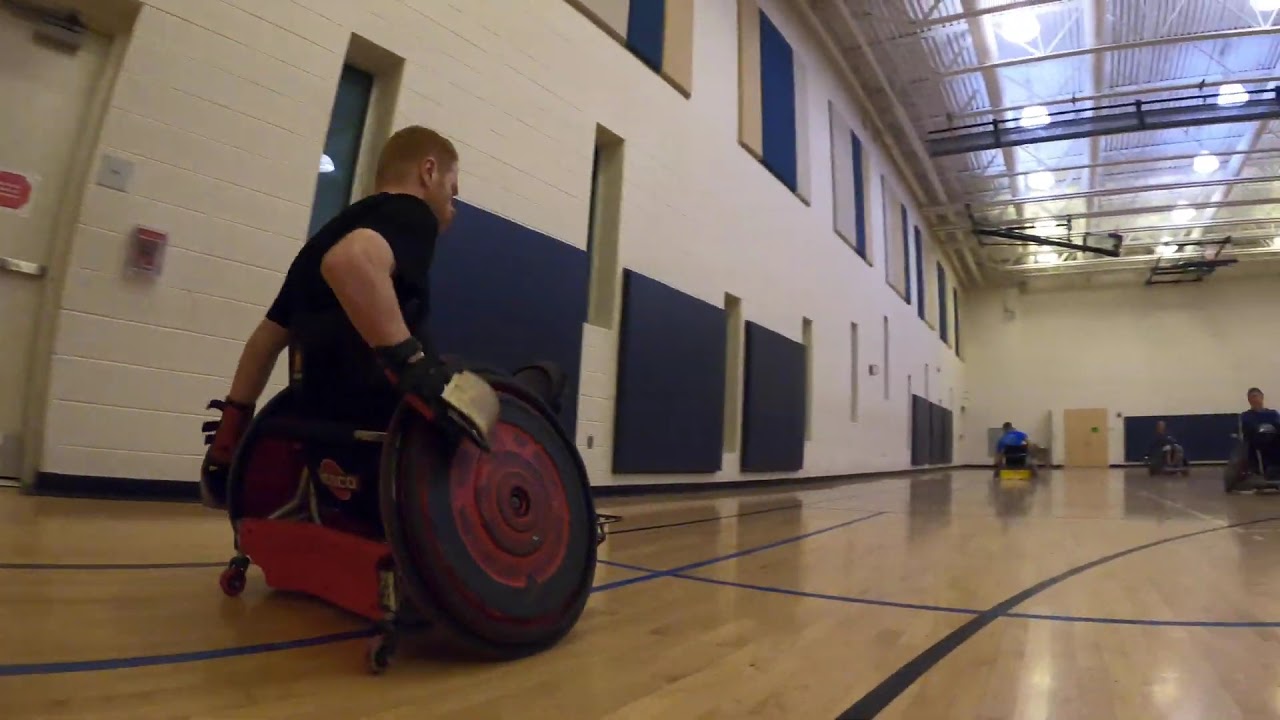The image captures a vibrant scene inside a large sports gymnasium with white cinder block walls, padding, and high ceilings adorned with incandescent lamps. The foreground prominently features a muscular man, likely in his late 20s, seated in a rugged red and black sports wheelchair with heavy-duty tires angled outward for agility and speed. His hands, one gloved, are positioned on the wheels, indicating movement down the gym floor. The gym's distinctive features include a folded-up basketball hoop, suggesting an alternative wheelchair sport in progress rather than basketball. In the background, three more men in wheelchairs can be seen, albeit at a distance, emphasizing the sense of action and competition in the atmosphere. The ceiling includes a section of glass panels, allowing light to filter through into the gym, enhancing the overall clarity and energy of the scene.